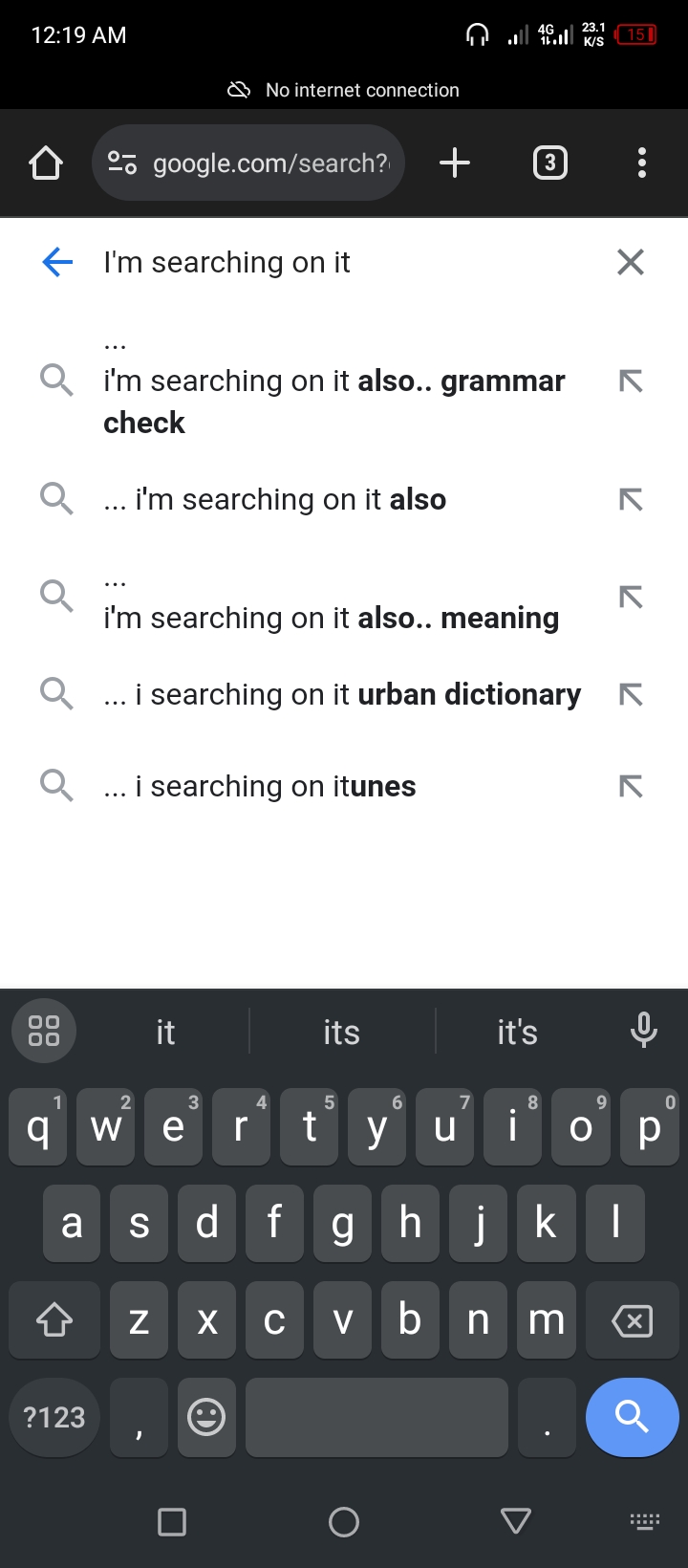This is a screenshot of a messaging application displayed on a smartphone. The phone features a black header and a black status bar. In the status bar, the top left corner shows the time as 12:19 AM, while the top right corner displays an icon of headphones and a red battery icon indicating a low charge at 15%. Below the status bar is an address bar with navigation buttons: a home button on the left, and a plus button on the right, indicating the option to open more tabs with a current total of three tabs open. The address bar also shows a "No internet connection" message.

Subsequent to the address bar is a white section. The first line of this section contains a general search field with an "X" icon on the far right. The listed search terms include "I'm searching on it," "I'm searching on it also grammar check," and "I'm searching on iTunes."

Below this white section is a black, QWERTY keyboard. The keyboard does not display the number line, which can be accessed by pressing the "?123" button located at the bottom left corner. On the bottom right corner of the keyboard is a blue search button, and the top right corner features a microphone icon.